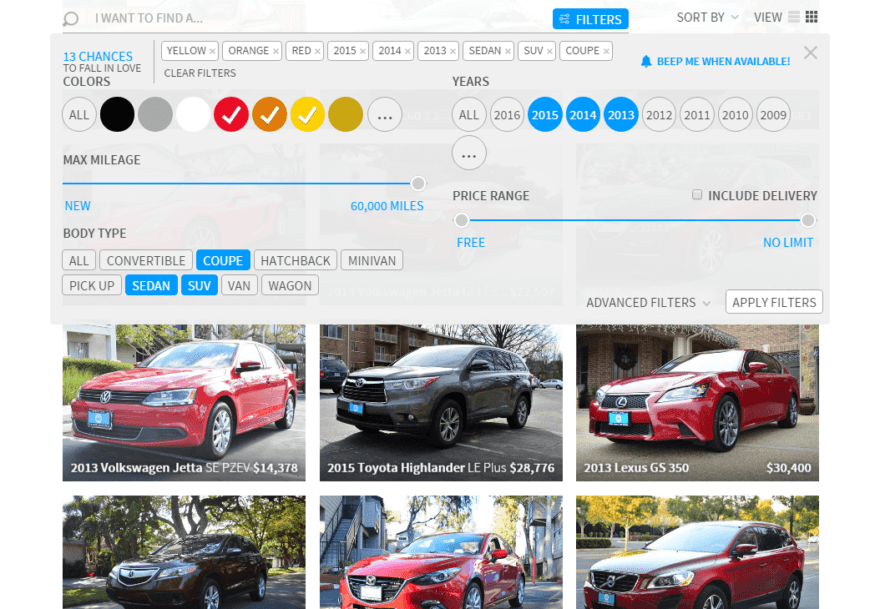The image displays a detailed section of a website focused on filtering search results for vehicles. 

At the top of the webpage, there's a small gray search bar featuring a magnifying glass icon with the placeholder text "I WANT TO FIND A..." in uppercase letters. To the right, there's a button labeled "FILTERS", displayed on a blue background with white uppercase text.

Next to the filters button, there's a "SORT BY" option with a drop-down menu, both in dark gray letters, followed by a "VIEW" option, also in dark gray uppercase letters.

The main content area features a light to medium gray background. In the top left corner, the text "13 CHANCES" is prominently displayed in blue. Directly below this, gray text reads "TO FALL IN LOVE WITH COLORS", all in uppercase. A horizontal line divides the sections.

Below this line, there are various filter options, including colors and years. Highlighted filters appear in blue for the years 2015, 2014, and 2013, while color filters for red, orange, and yellow have white checkmarks.

The "CLEAR FILTERS" option is also present. To the side, there's a notification option "NOTIFY ME WHEN AVAILABLE" accompanied by a bell icon, both displayed in blue text.

Beneath this, circular color filters appear for black, gray, white, red, orange, yellow (with white checkmarks), and a circle with three dots representing additional options. Year filters are listed from 2016 down to 2009, with 2015, 2014, and 2013 highlighted in blue, and an additional circle with three dots indicating more options.

Further down, there are input settings for "MAX MILEAGE" showing new to 60,000 miles, "PRICE RANGE" with options including "INCLUDE DELIVERY" and "FREE NO LIMIT". Multiple vehicle types are also selectable (e.g., convertible, coupe, hatchback, minivan, pickup, sedan, SUV, van, wagon). Several vehicle categories such as coupe, sedan, and SUV have been chosen.

Lastly, the page showcases six different vehicles available for selection based on the applied filters.